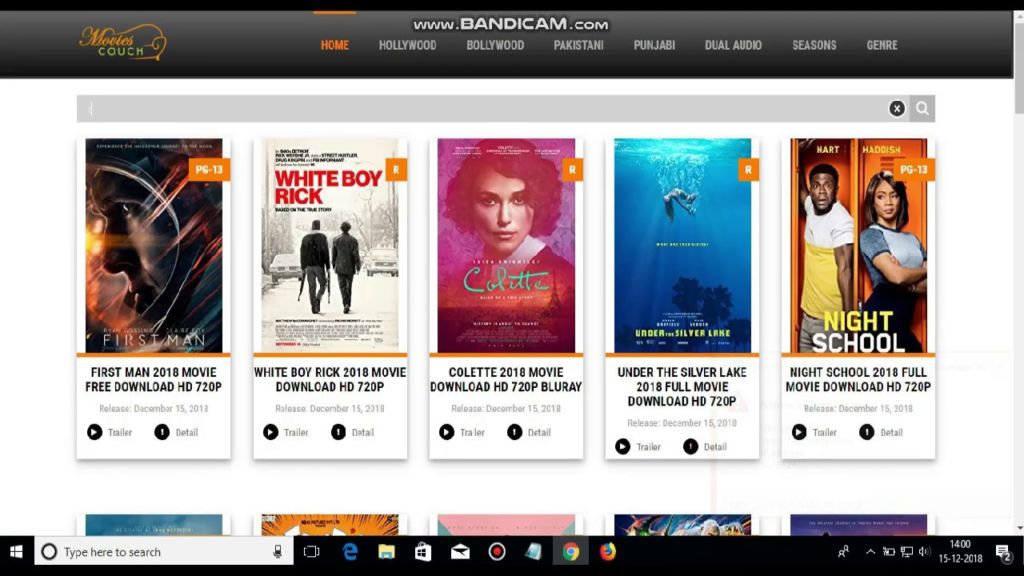This is an image from the website www.bandacam.com, featuring a banner on the left-hand side that reads "Movies Couch." An orange "Home" button is prominently displayed, followed by a menu listing various categories: Hollywood, Bollywood, Pakistani, Punjabi, Dual Audio, Seasons, and Genre. 

Below the banner, there is a list of five different movies, each showcased with a distinct cover image and title:

1. **First Man (PG-13)**: The cover features a man looking contemplative, set against a background filled with stars.
2. **White Boy Rick**: This black-and-white cover displays two men walking away, with cars and snow-covered trees in the background.
3. **Colette**: The image shows a woman with short, somewhat curly hair, looking directly at the camera. She is wearing a white collared outfit.
4. **Under the Silver Lake**: This cover depicts a person with long hair falling upside down into water, with a striking blue background.
5. **Night School**: The image features two characters: a black man seemingly trapped inside a locker and a woman standing beside him with her arms crossed.

At the bottom of the image, various website icons are displayed, adding to the navigational options for users.